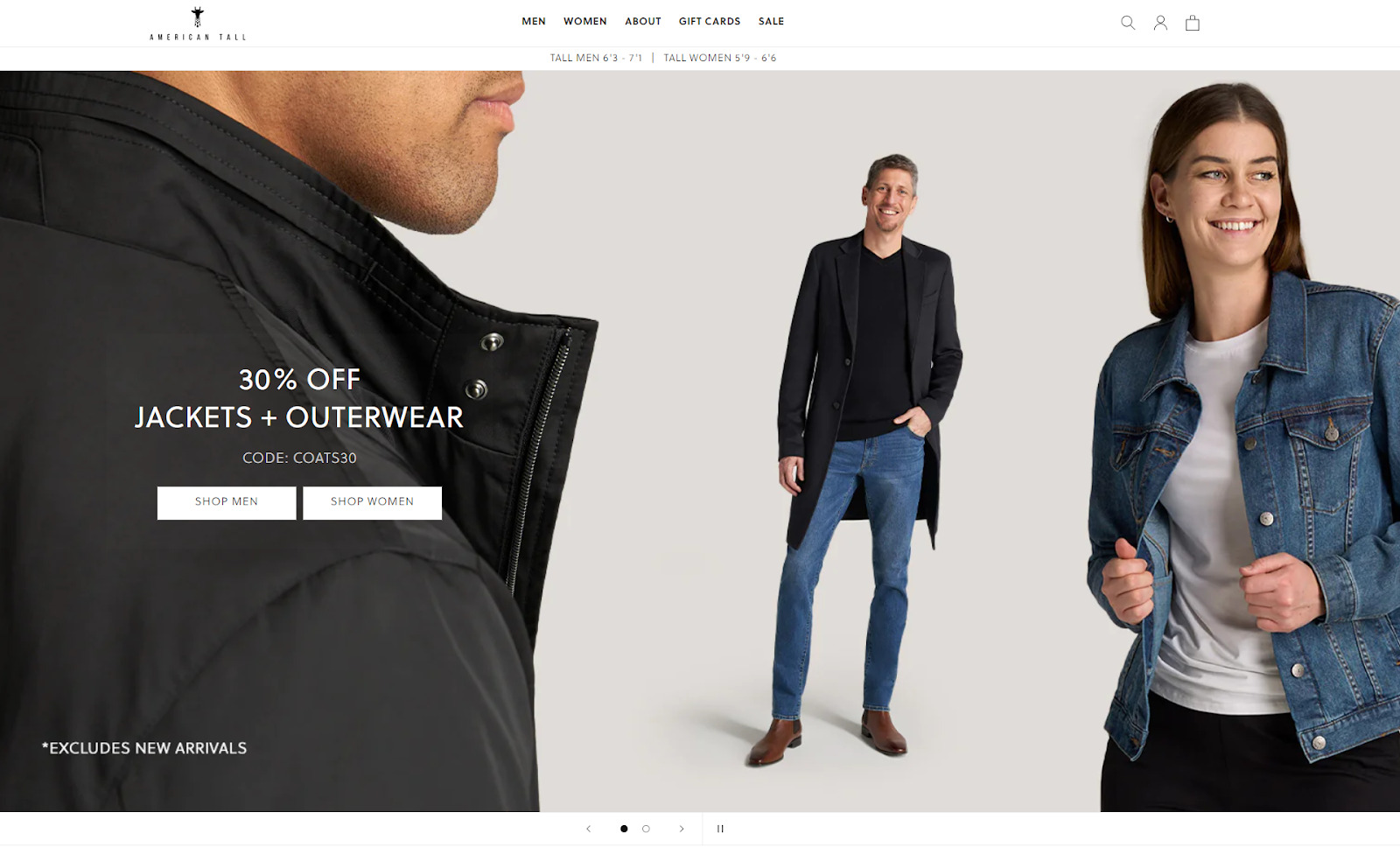The image appears to be a screenshot from a clothing website named "American Tall," as indicated by the small logo and name located in the upper left-hand corner. Centered at the top of the page is a menu featuring categories such as "Men," "Women," "About," "Gift Cards," and "Sale." Toward the upper right-hand side, three faint icons are visible, though their exact details are indistinguishable due to their light hue.

Just beneath this navigation area, text denotes "Tall Men" followed by a slash and then "Tall Women." The primary visual element of the image is a large photograph occupying most of the page. On the left-hand side of this photograph, a man is pictured in a close-up shot, turned to the right. The close-up nature of the image results in his head being partially cut off at the top, with a clear view of his right shoulder and the right side of his face. In the background, another man can be seen, adding depth to the photograph.